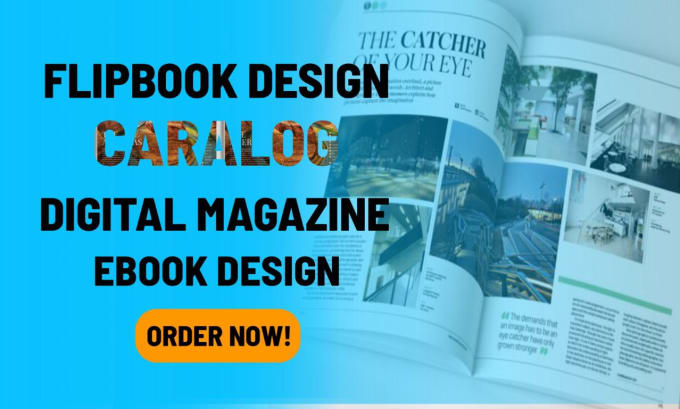This advertisement features a light blue background with a gradient that fades into a transparent section, revealing an open booklet beneath it. The left side of the ad prominently displays several text elements in different styles and colors. At the top, bold black text proclaims "Flip Book Design," followed by a colorful, magazine-style cutout text that reads "Carologue." Directly below, in another bold black font, the text states "Digital Magazine" and "E-Book Design." An orange call-to-action button at the bottom urges viewers to "Order Now!" in black text with an exclamation mark.

On the right side of the ad, there is a semi-transparent open booklet. The main headline within the booklet reads "The Catcher of Your Eye." The booklet's pages display a grid layout featuring various images of city structures, imitating a realistic digital magazine spread. The booklet includes additional text that is too small to read but suggests further content within the digital magazine being advertised. This visually compelling ad appears designed for online platforms, enticing users to explore and purchase the digital magazine.